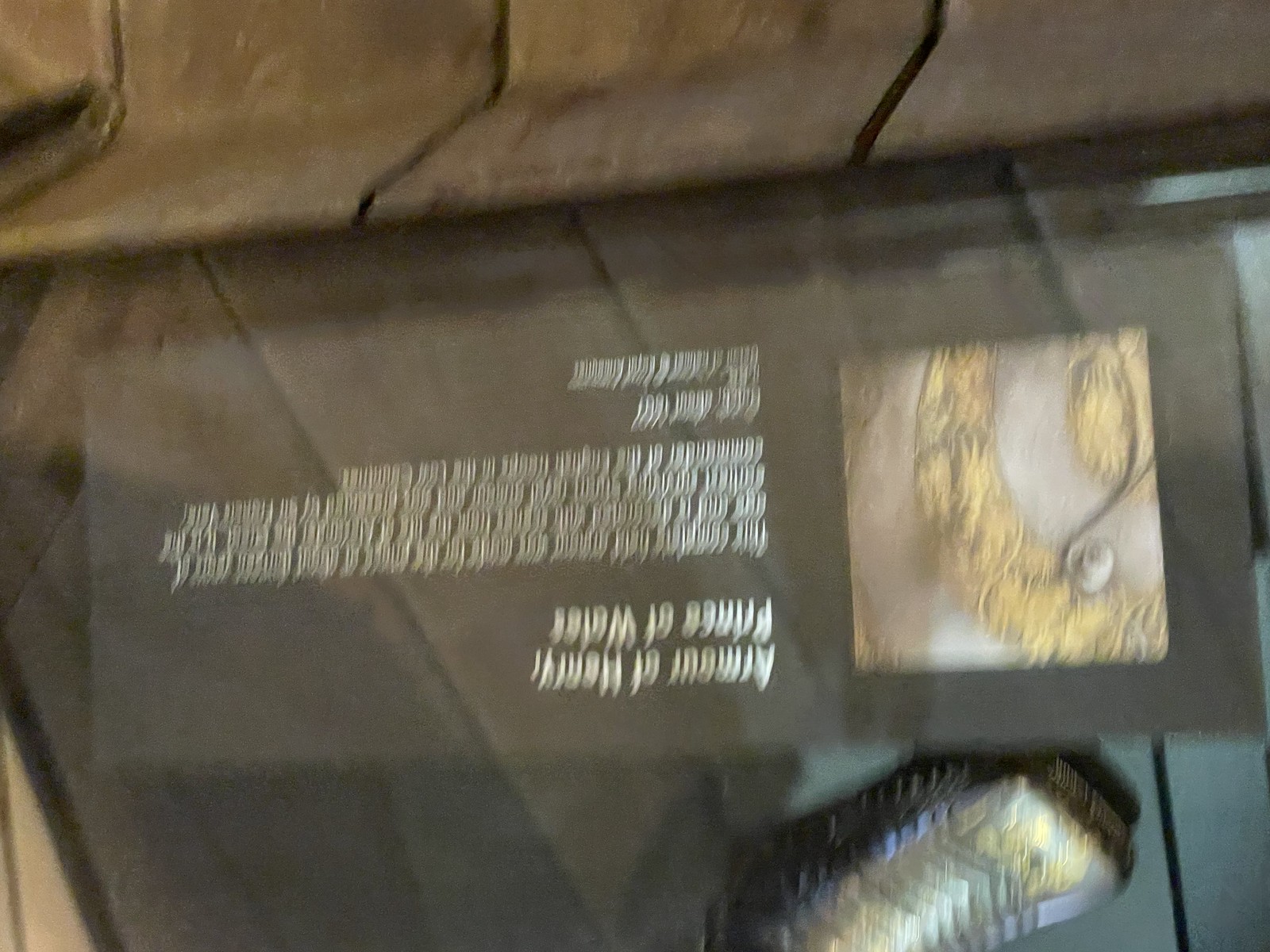This image captures an inverted view of a museum display featuring the "Armor of Henry, Prince of Wales." The photograph suffers from significant camera shake and motion blur, making details challenging to discern. On the left side of the display, there is a placard with a title readable as "Armor of Henry, Prince of Wales." Below the title, a large block of white text is present, though it is illegible due to the blurriness. On the right side, there is a close-up image that likely showcases a specific detail of the armor. The armor itself is faintly visible at the bottom of the frame. The disorienting perspective and motion blur heavily obscure the exhibit's finer details.